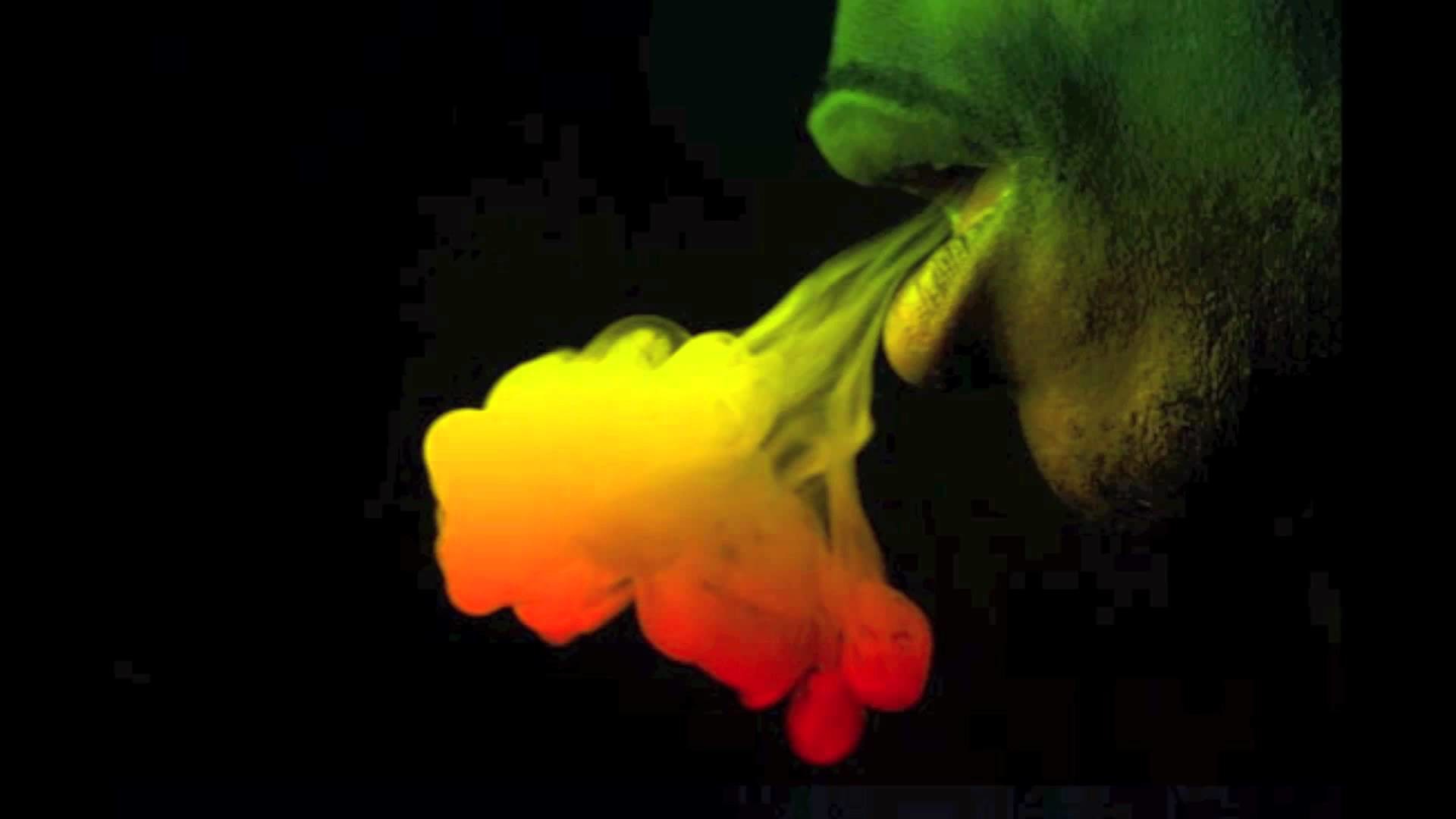The image depicts a dark-skinned male with a close-cropped mustache and raggedy stubble blowing smoke from his slightly open mouth. The composition focuses on the lower part of his face, primarily showing his chin, mouth, and a portion of the cheek, with a distinctive green and yellow tint on his skin. The smoke - a mix of yellow, red, and orange hues - billows out in a dense cluster at the center of the horizontal, rectangular image, set against a stark black background. The man's mouth is positioned in the top right corner, oriented downward toward the middle of the frame. The overall color scheme of the image, featuring gradients of green, yellow, and red, evokes an Afrocentric aesthetic reminiscent of Bob Marley.